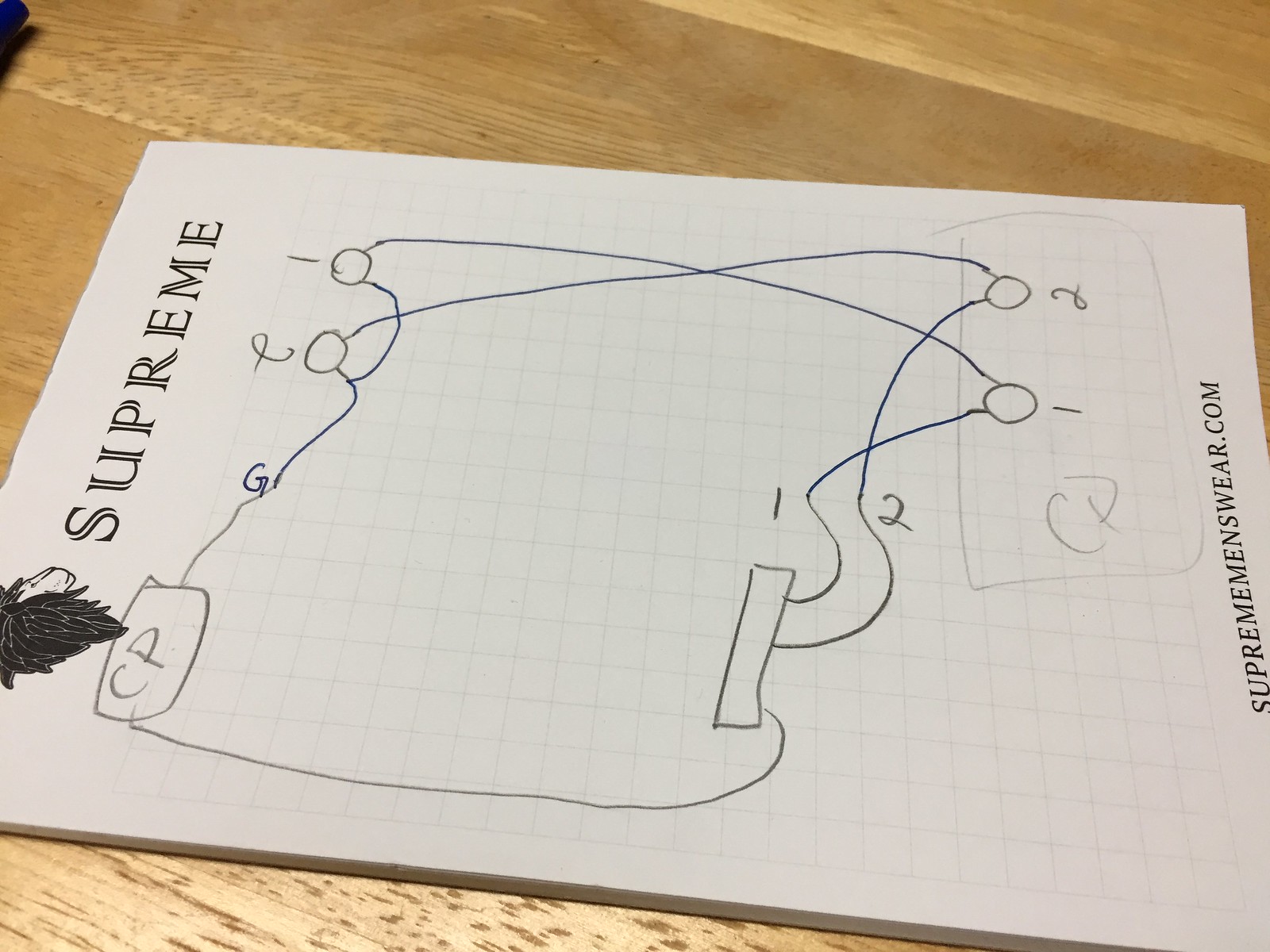A top-down shot of a notepad on a wooden table features a detailed engineering diagram. On the left side of the paper, "Supreme" is prominently written at the top, followed by the Supreme lion logo at the bottom. A series of technical sketches occupy the center, with diagrammatic lines and annotations. Specifically, the bottom left corner highlights a small square labeled "CP." Blue pen marks point upwards to "Figure G." At the top of the diagram, two numbered circles, 1 and 2, connect to corresponding figures on the right side of the paper. Another "CP" within a square is situated on the right side, while the bottom right corner bears the text "suprememenswear.com." The diagram is sketched on grid paper, enhancing its technical feel.